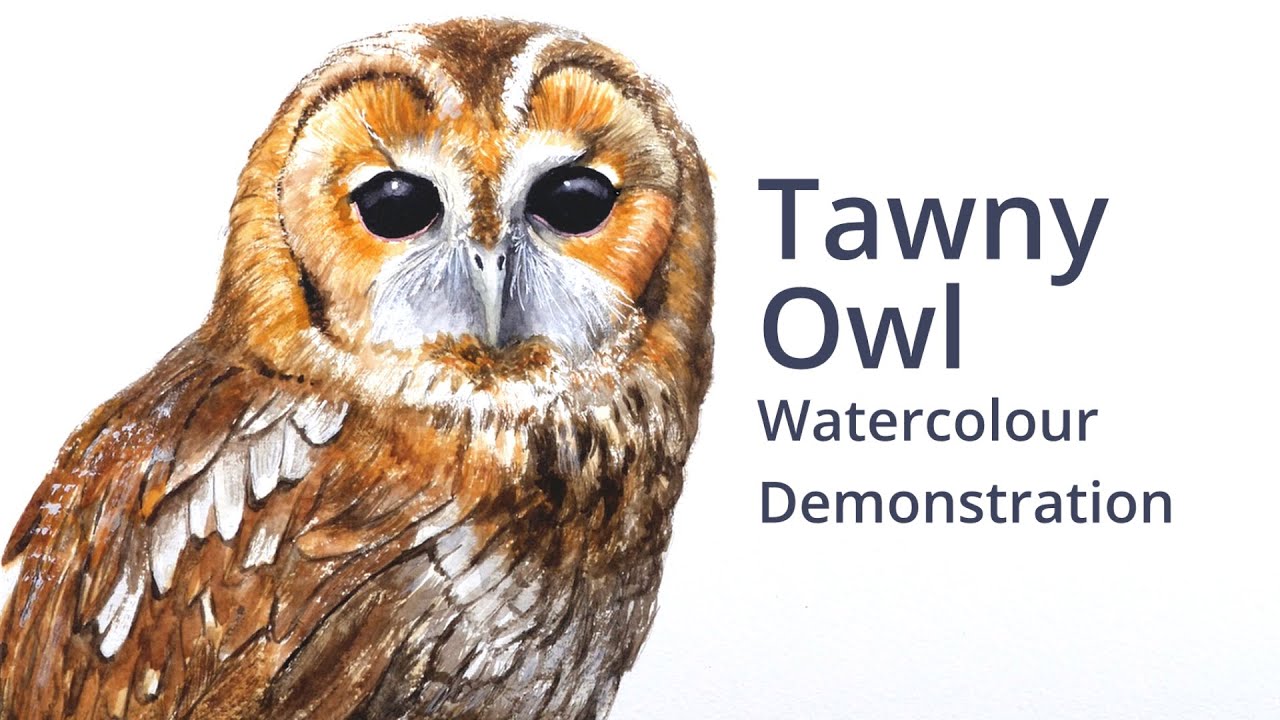The image showcases a detailed watercolor drawing of a tawny owl on the left side against a solid white background. The tawny owl's head is turned towards the viewer, displaying its striking black eyes with small white reflections. Its beak is predominantly white with some grayish hues and white spots for the nostrils. The owl's face features a mix of orange, white, and gray around the eyes, creating a vivid contrast. The upper part of the owl's head and body is brown, with a transition to lighter brown and white dabs towards the neck and lower body. The wings are brown and appear to be resting together. White feathers also accent the ends of its wings and under its beak.

To the right of the owl is the text in a thick black font that reads "Tawny Owl" in large letters, followed by "Watercolor Demonstration" in smaller text underneath. The word "Watercolor" is spelled in the British style as "W-A-T-E-R-C-O-L-O-U-R." The overall presentation suggests a realistic and detailed demo of the tawny owl art piece.